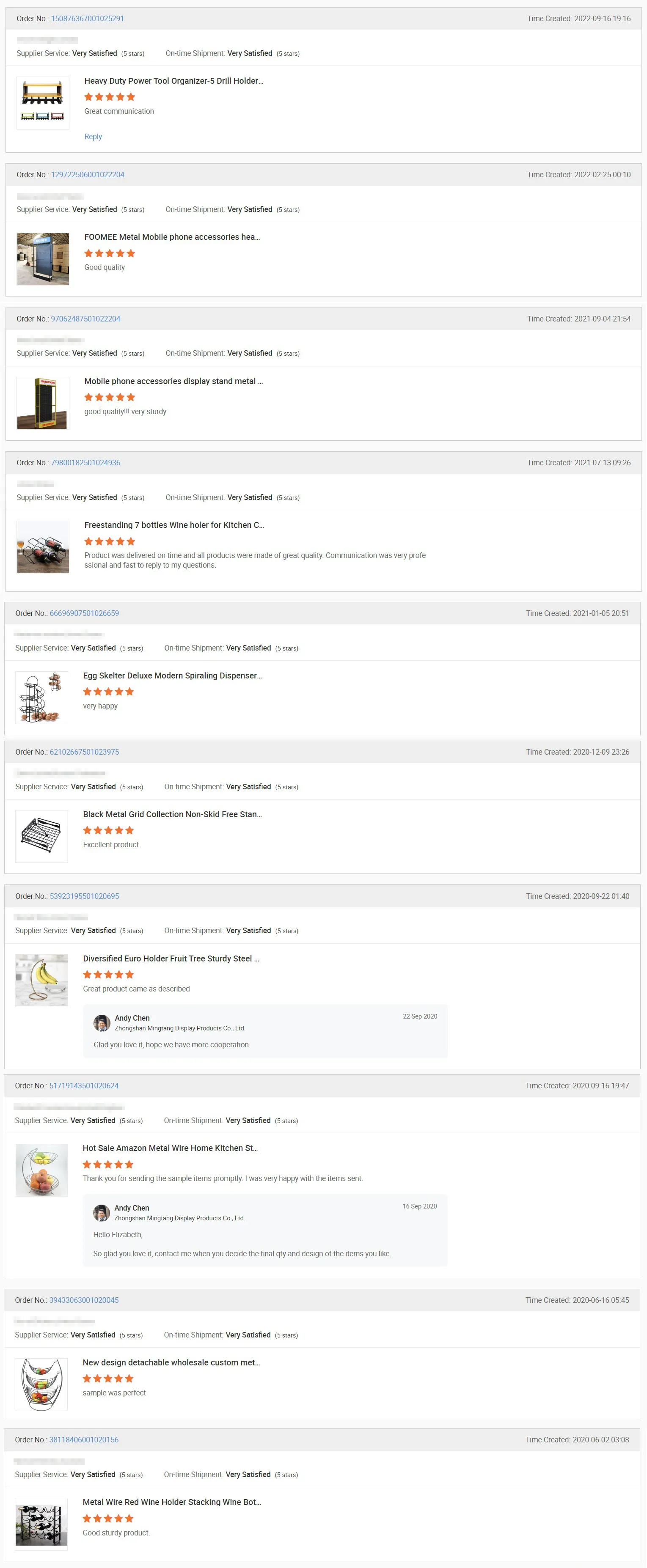The image showcases a column of ten Amazon.com reviews, each arranged in a uniform format. Every review features an order number in blue text situated in the top left corner of its box, while a time stamp is displayed in the top right. Below, product details are written in black text. On the center left, each review includes a small, somewhat blurry image of the corresponding product. To the right of the image, the product name is displayed, followed by a star rating and a brief, partially legible user review. A blue link is present at the bottom of each review.

The products reviewed appear to be diverse and include: a painting set as the first item, a blue screen for the second, a cabinet for the third, and more painting supplies for the fourth. The fifth item resembles a coffee pad holder, while the sixth looks like a grill. The seventh item appears to be banana art, the eighth a food plate, the ninth a fruit holder, and the tenth looks like a dumbbell holder for a gym. The text and images are small and somewhat indistinct, making it difficult to discern specific details.